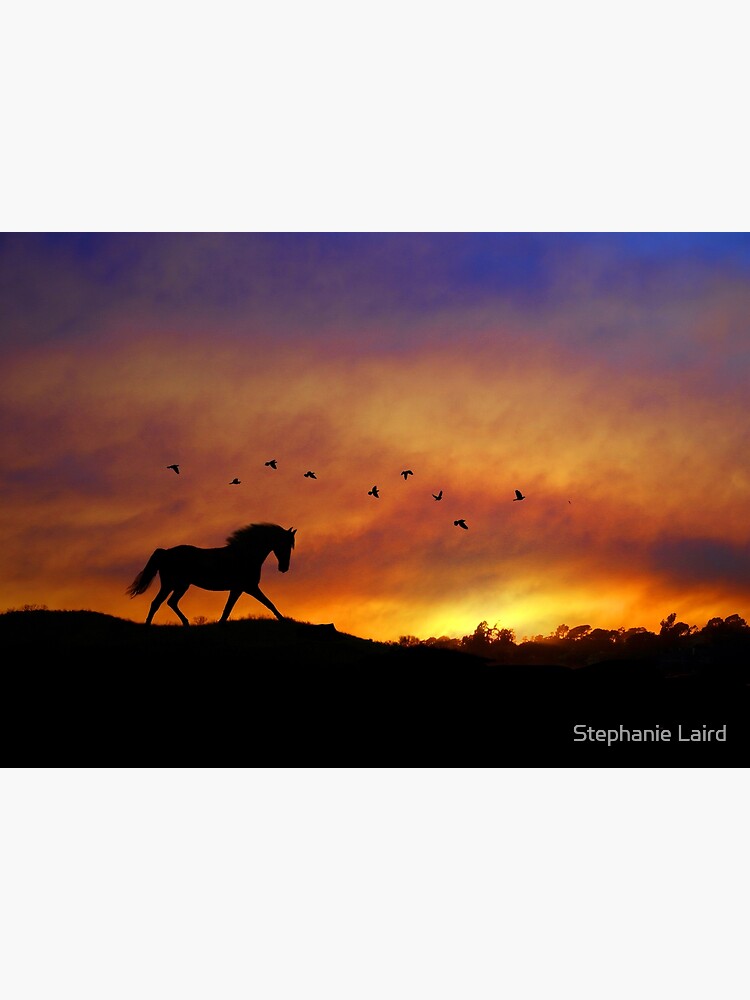This captivating calendar-like image by Stephanie Laird features a striking silhouette of a horse walking along the ridge of a hill at sunset. The landscape and horse are rendered in deep black, creating a stark contrast against the vibrant sunset sky. Positioned slightly left of center, the horse is moving toward the right side of the image. Above the horse, a small flock of nine birds also appears in silhouette. The sky showcases impressive hues, transitioning from intense red, yellow, and orange near the horizon to darker shades and even a hint of purple at the top. There is a touch of white mist or fog blending with the vibrant clouds. The photographer's name, Stephanie Laird, is prominently displayed in white text in the bottom right corner, completing this breathtaking scene.